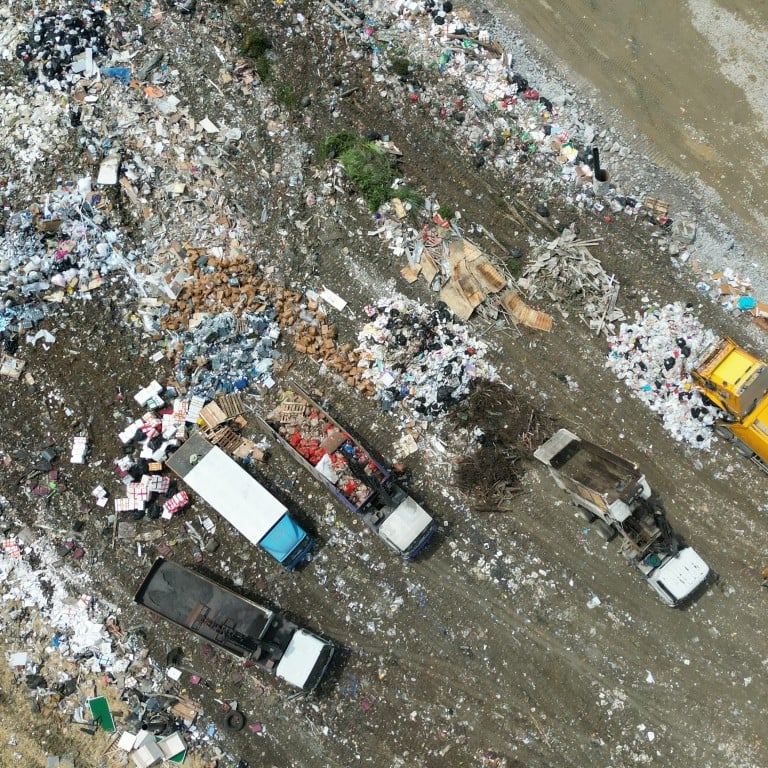This is an aerial view, taken from a drone or helicopter at an altitude of at least 100 feet, of a sprawling landfill site characterized by various piles of trash and refuse. The scene is dominated by five older trucks, each of a different color—yellow, white, black, blue—parking and dumping their loads onto the mixed rubble and dirt below. One truck has its bed lifted, actively unloading its contents onto the ground. The area is littered with diverse piles, some resembling boxes, others appearing as general trash or debris, creating an overall impression of neglect and decay.

Tire tracks from the trucks lead towards the bottom-right corner of the image, suggesting a systematic dumping operation, though several trucks appear worn out and possibly non-operational. Among the scattered debris, there are noticeable items such as glass, plastic bags, and black trash bags grouped in the top left corner. The landfill also features areas of barren dirt interspersed with small patches of greenery. Different types of waste appear to be segregated, with piles of industrial debris, household trash, mulch, compost-like material, wood, and rocks spread across the site, indicating organized dumping practices based on waste type. In the distance, emptier sections of the landfill, devoid of refuse, mark zones awaiting future use or those recently cleared.